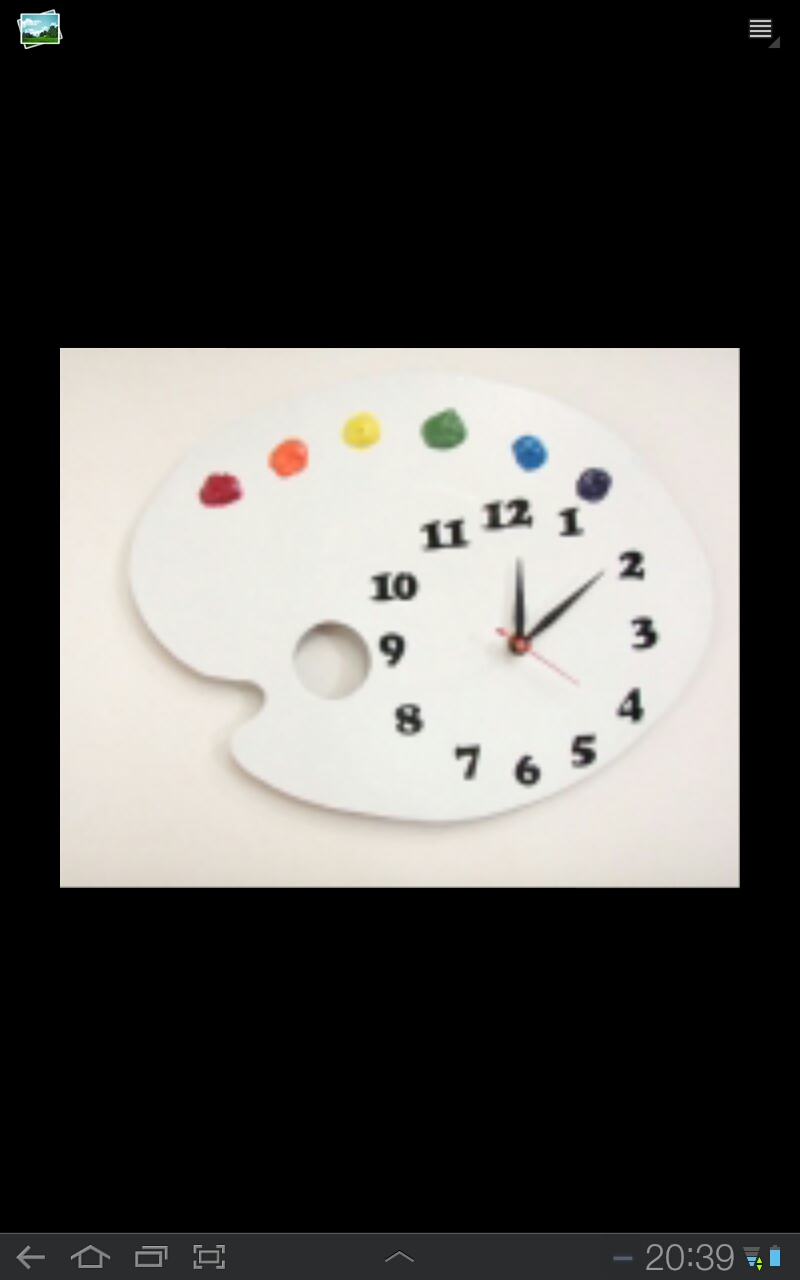This screenshot appears to be from a smartphone or tablet, displaying a screensaver against a completely black background. Prominently centered is a white artist's palette, which doubles as a clock. On the palette, black numerals are positioned around the edge like a traditional clock, with black hour and minute hands and a red second hand indicating the time. Lined along the top edge of the palette are dollops of paint in a spectrum of colors: red, orange, yellow, green, blue, and indigo (or violet). Additionally, at the very bottom of the screen are various phone icons and a widget displaying "20:39." In the upper left-hand corner of the screen is a small icon featuring a blue sky, some clouds, grass on the ground, and trees in the background, possibly part of the device's interface. This detailed composition combines both artistic and functional elements, blending the creative imagery of a painter’s palette with the practical use of a clock.